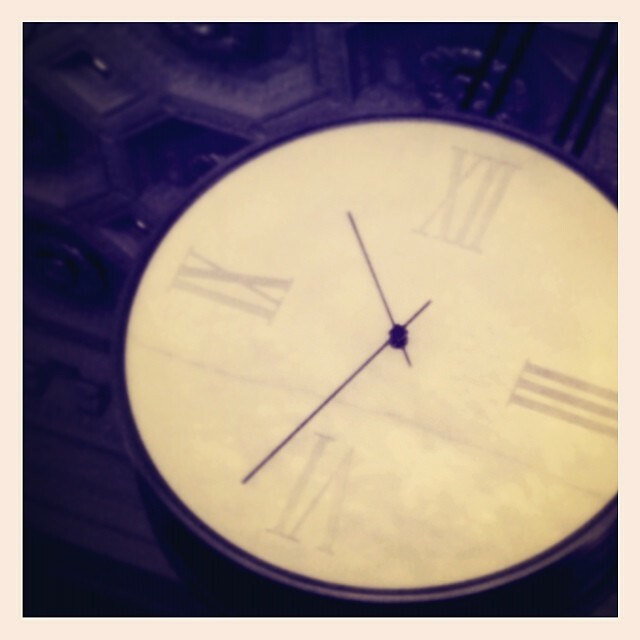A meticulously crafted, computer-generated artwork or a heavily edited photograph, this image predominantly showcases a clock face, reminiscent of the serene, cratered surface of the moon, cloaked in a muted off-white hue. Encircled by a substantial, off-white border, the timepiece features elegantly classic Roman numerals that evoke a bygone era. The hour and minute hands, resembling slender black needles, stand in stark contrast against the pale face. Surrounding the clock, a mysterious and shadowy dark blue-purple background hints at the ghostly silhouettes of indistinguishable buildings, adding an enigmatic and almost ethereal ambiance to the overall composition.